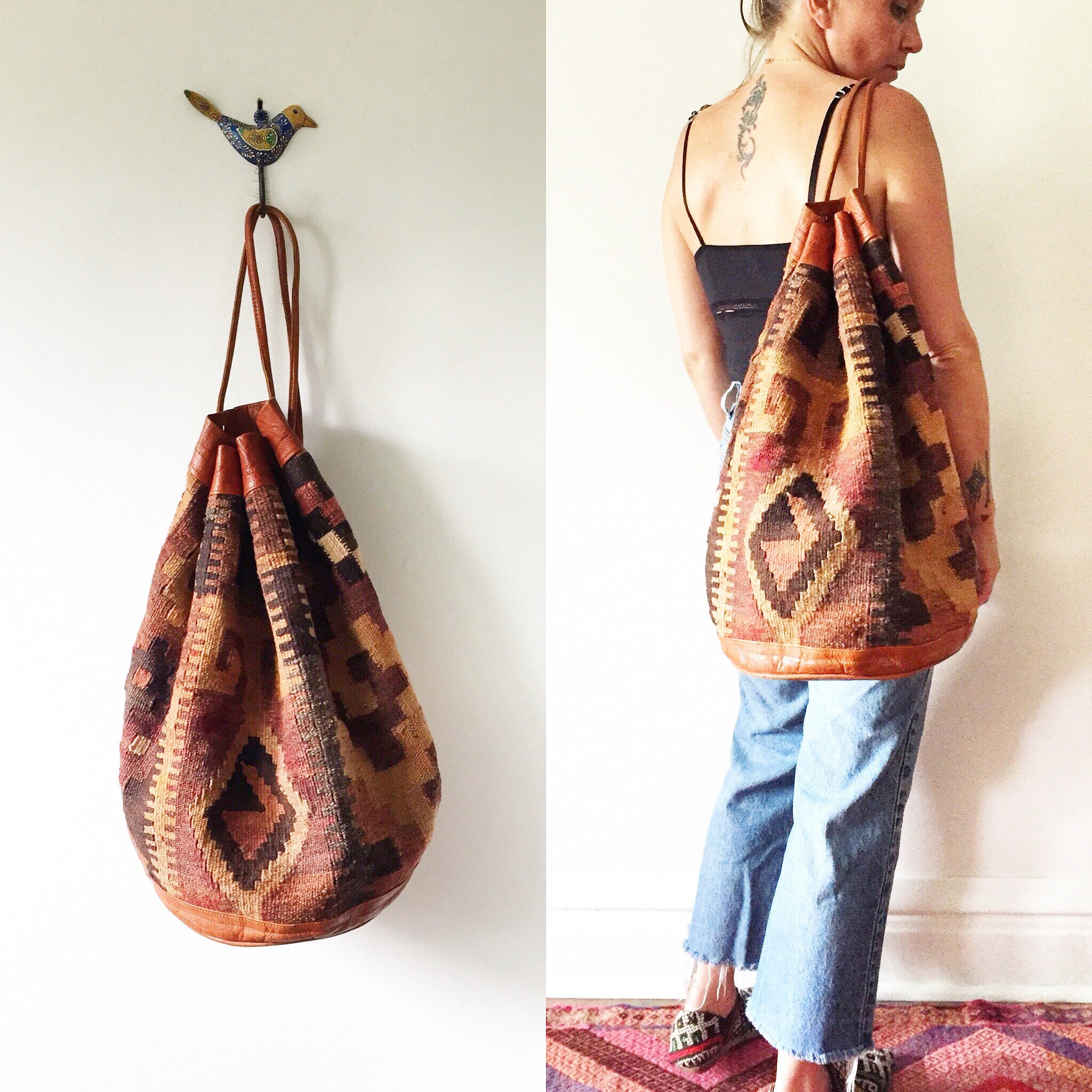The image is a vertically aligned diptych with two photographs side by side, set indoors against a white wall. On the left, a brown hobo bag with intricate patterns of diamonds, rectangles, and squares in various shades of brown and black hangs from a decorative bird-shaped hook attached to the wall. The bird hook is oriented with its tail to the left and its beak to the right. On the right, a young, light-skinned blonde woman is seen from behind, turned in profile. She has a prominent tattoo running down the center of her back and another on her left wrist. She is dressed in a black spaghetti-strap camisole, blue jeans with frayed edges, and black and white canvas loafers. She carries the same patterned hobo bag on her right shoulder. Her hair is styled up, revealing her bare shoulders and arms. She stands on a colorful carpet featuring a vivid pattern of diamonds in purples, reds, and pinks. The juxtaposition of the images effectively showcases the bag's design both hanging on the wall and worn by a person.